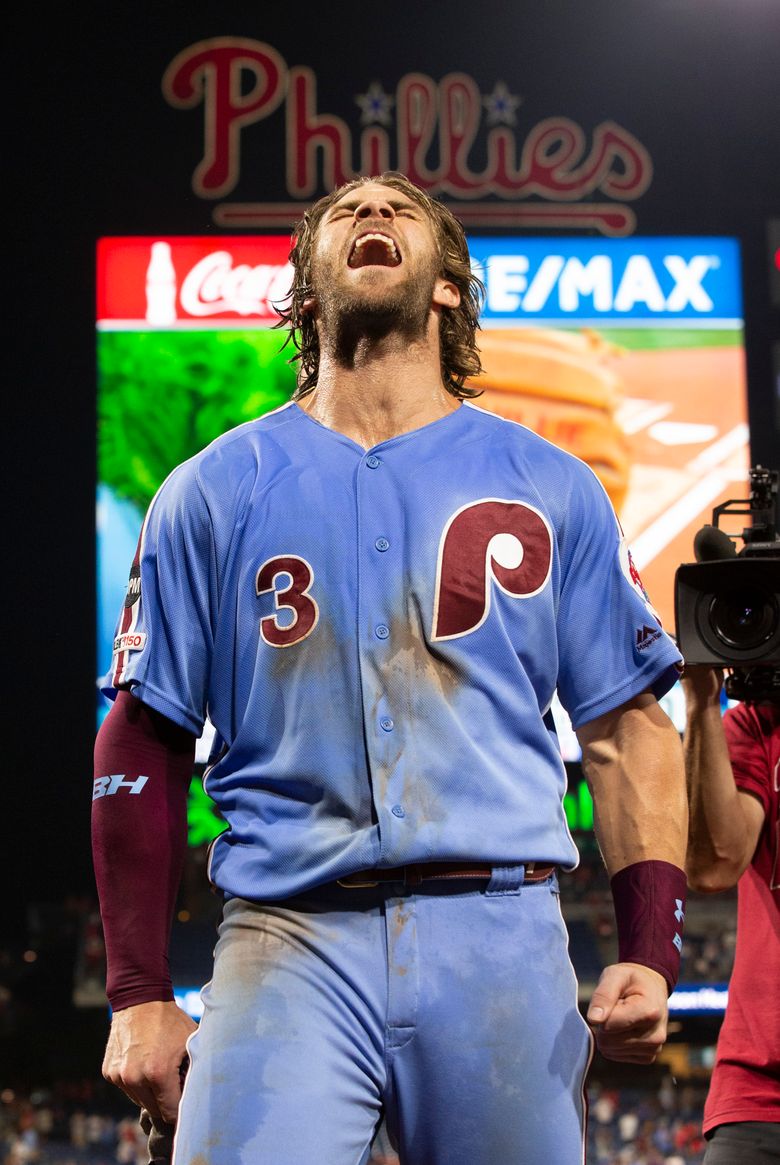In this celebratory image, a baseball player, clad in a light blue and burgundy uniform, commands attention. This athlete, representing the Phillies, prominently sports the number 3 and the letter P in maroon on his dirt-smeared jersey. His appearance is highlighted by wet, scraggly hair and intense facial expression - mouth wide open and eyes closed, as he tilts his head upwards in a roar of victory. His right arm features a protective dark maroon sleeve, and a matching band adorns his left wrist. A cameraman, dressed in a red shirt, captures the triumphant moment from the player's side. The backdrop features a Megatron LED board, with a Phillies header and a Coca-Cola advertisement, further situating this scene within an electrifying stadium atmosphere.